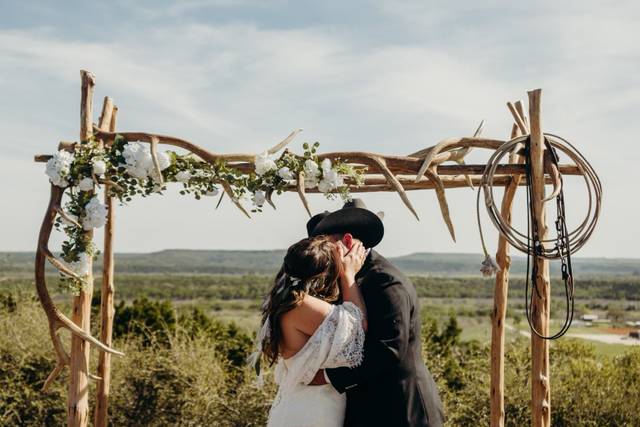The image depicts a vibrant and picturesque outdoor wedding scene, framed by a clear blue sky dotted with white clouds. In the background, a rolling landscape of grassy hills and fields, interspersed with patches of brown dirt or sand, stretches out beneath the azure sky. To the right side, puddles of reflective blue water add a touch of serenity to the scene.

Dominating the foreground are masses of overgrown bushes and grass, with paler green foliage in the front and richer green bushes slightly further back. Positioned centrally in the middle of the image are a man and a woman, locked in a tender kiss, suggesting they have just been married. The man, dressed in a black suit and black cowboy hat, embraces the woman, whose white dress and matching hair accessory signal her role as the bride.

Behind the couple, the altar is a rustic construction made from brown sticks, logs, and deer antlers, adorned with white flowers and green leaves. To the right of the altar hangs a lasso, a brown rope with a black whip attached, adding to the rustic, Western motif. A third person, likely the officiant, is partially visible behind the couple, marked by the distinctive presence of a gray cowboy hat.

This beautifully bright, sunny day captures the joyous moment of a newlywed couple's first kiss against the scenic backdrop of a distant mountain range, which lies bathed in the perfect light of the wedding day.